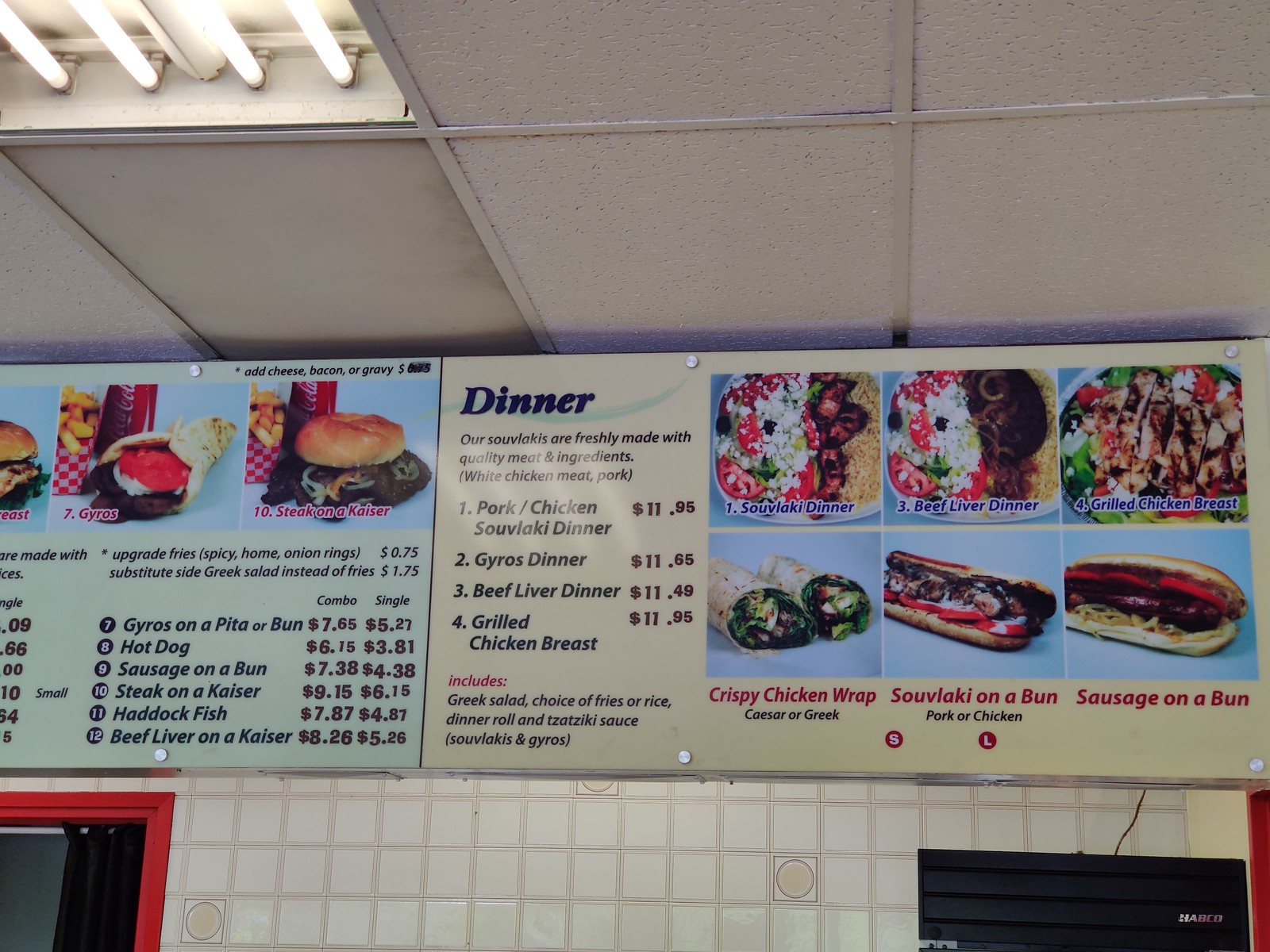This image showcases the interior of a diner, captured from a high angle. The ceiling is a creamy white color, adorned with ceiling lights in the top left corner. Below, a large menu board prominently displays various food options, accentuated by pictures of fresh fries, Coca-Cola, and burgers. 

The menu highlights several items labeled in red letters: number 7 "GYROS," and number 10 "STEAK ON A KAISAR." Above these, in black text, it reads "Add cheese, bacon, or gravy." Further down, it offers additional options to upgrade to spicy fries, home fries, or onion rings for $0.75, or substitute with a side Greek salad for $1.75. The menu also distinguishes between combos and singles with a mix of black and red text.

On the right side of the board, the word "Diner" is displayed in bold blue letters. Although some text is obscured by a flashing light, below it, detailed listings of meal options are visible:

- Number 1: "SOUVLAK Dinner" in blue text.
- Number 2: "Beef/Liver Dinner."
- Number 3: "Grilled Chicken Breast," depicted with a brown, grilled chicken breast and salad.
- Number 6: "Crispy Chicken Wrap" with options for Caesar or Greek style, shown wrapped.

Further down the menu, items such as "Slow Funky on a Bun," with options for pork or chicken, and "Sausage on a Bun" are listed. The initial letters "S" and "L" are visible, likely indicative of small and large sizes for these items.

The overall ambiance suggests a classic, perhaps family-owned diner with a varied menu offering both traditional and Greek-inspired dishes.